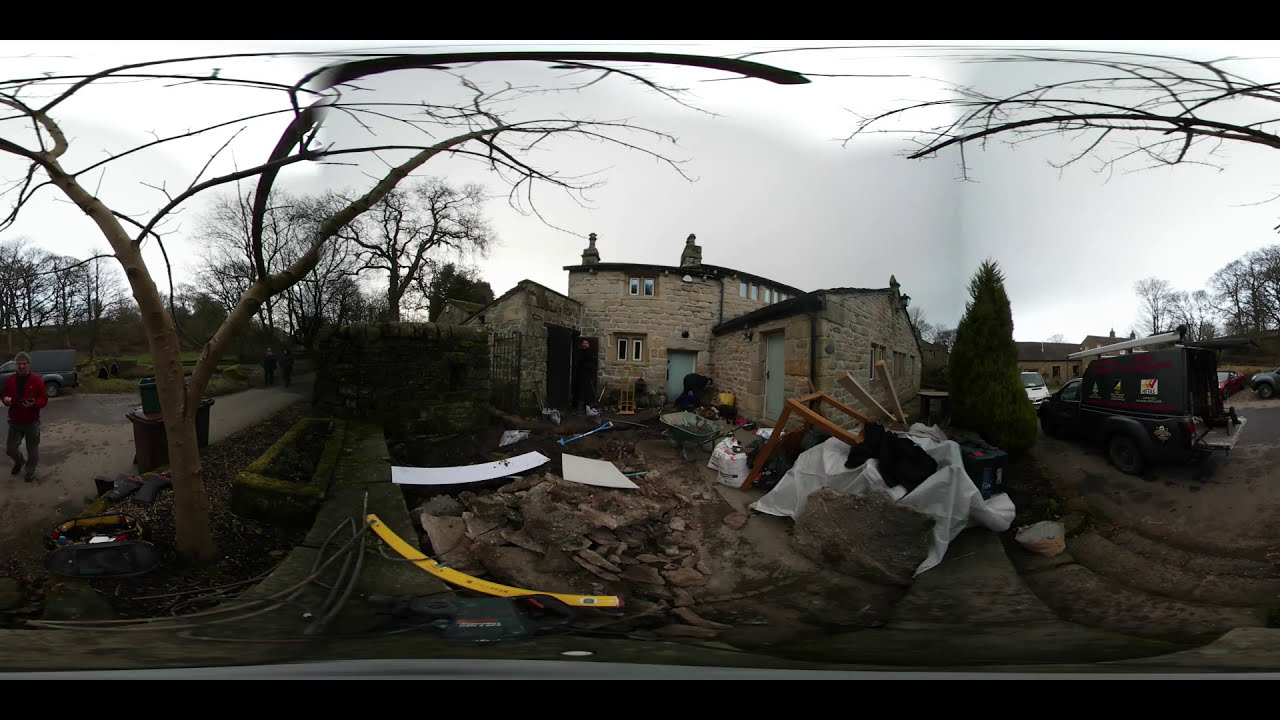The distorted panorama photograph shows a construction site centered around a light gray building composed of rocks and bricks. The photograph, framed with solid black borders on the top and bottom, gives an impression of a wide rectangular format. The building has two stories, with two small windows at the top and two more at the bottom. A flat roof covers the structure, which features a white door on the main building and another door on a right-side extension made of the same material. Directly in front of the building are piles of trash, sand, dirt, broken rocks, and wood, some covered with plastic. On the right side, pieces of wood stick up, while a dead tree with branches extending to the left and right stands prominently on the left. Additionally, there is a strip of a yellow bar and some white panels lying flat on the ground to the left. On the far left, a person wearing a red shirt and blue jeans is visible. Surrounding the scene are various trees, including a tall, dark green tree resembling a Christmas tree on the right. The background sky is filled with gray and white clouds, creating an overcast atmosphere. The image captures a moment in an outdoor, possibly residential neighborhood undergoing construction.